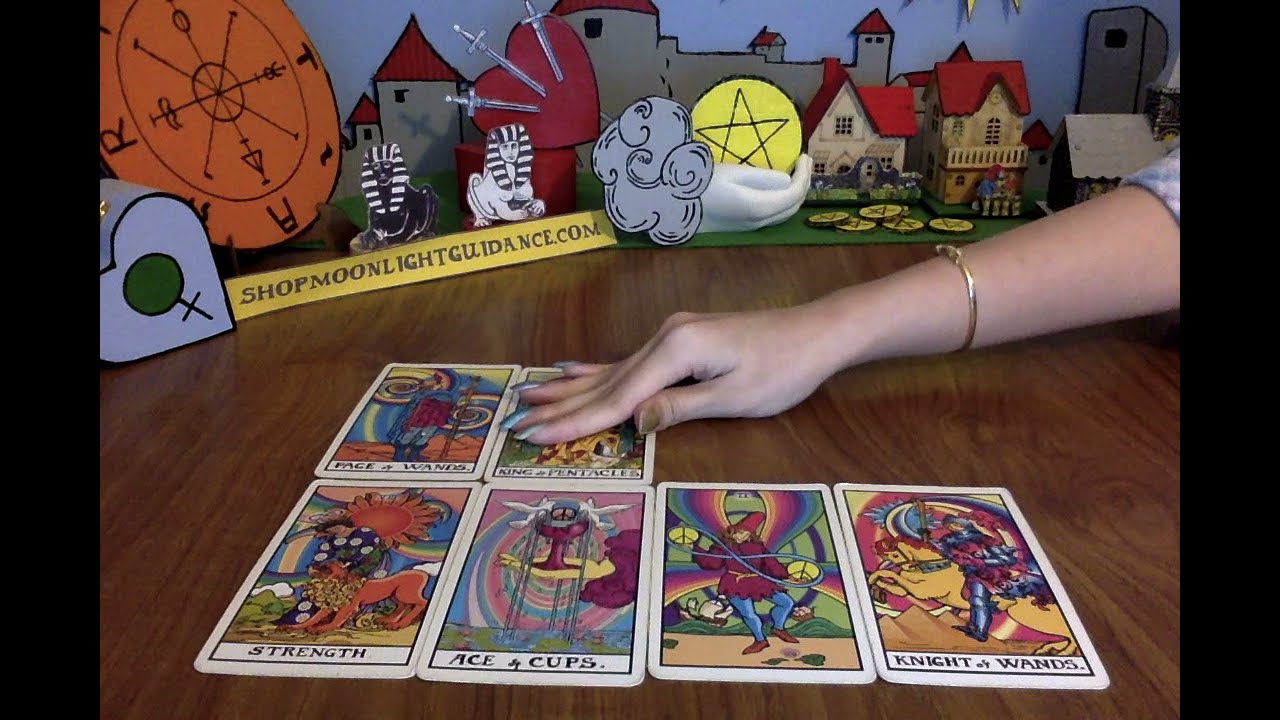The image depicts a set of colorful, tarot-like game cards arranged on a shiny wooden table. The cards are about half the size of a hand and are organized in two rows: four on the bottom and two on top. Some of the visible cards include ones labeled "Strength," "Ace of Cups," "Knight of Wands," and one without any text. The cards feature vibrant, cartoony illustrations in shades of orange, purple, blue, yellow, and green, depicting whimsical characters possibly related to the game they belong to.

A female hand with light blue painted nails, except for a thumb that is painted brown or discolored, reaches in from the right side of the image and touches one of the top row cards. The hand also has a bracelet on the wrist.

In the background, a cardboard wall displays an artistic mural featuring a medieval castle under a night sky with a grassy field in the foreground. Various occult-like symbols and decorated coins with black stars can be seen near the mural. On a yellow strip of paper in the upper left corner, the text "ShopMoonlightGuidance.com" is prominently displayed, suggesting that these tarot-like cards might be available for purchase through the website.